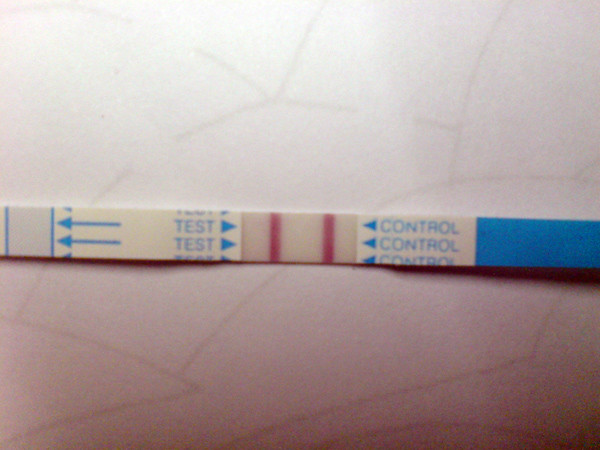The image depicts a test strip set against a marbled white and gray background. The strip features multiple indicators:

1. On the left side, blue arrows point toward a blue line area labeled "Test."
2. To the right of this, a segment marked with blue triangles directs attention to the center where a red line is visible.
3. Further to the right, the section labeled "Control" shows blue triangles indicating a red strip.
4. On the far right side, there's a noticeable blue strip.

Overall, the strip is a detailed design indicating specific test and control areas with corresponding blue and red markers.